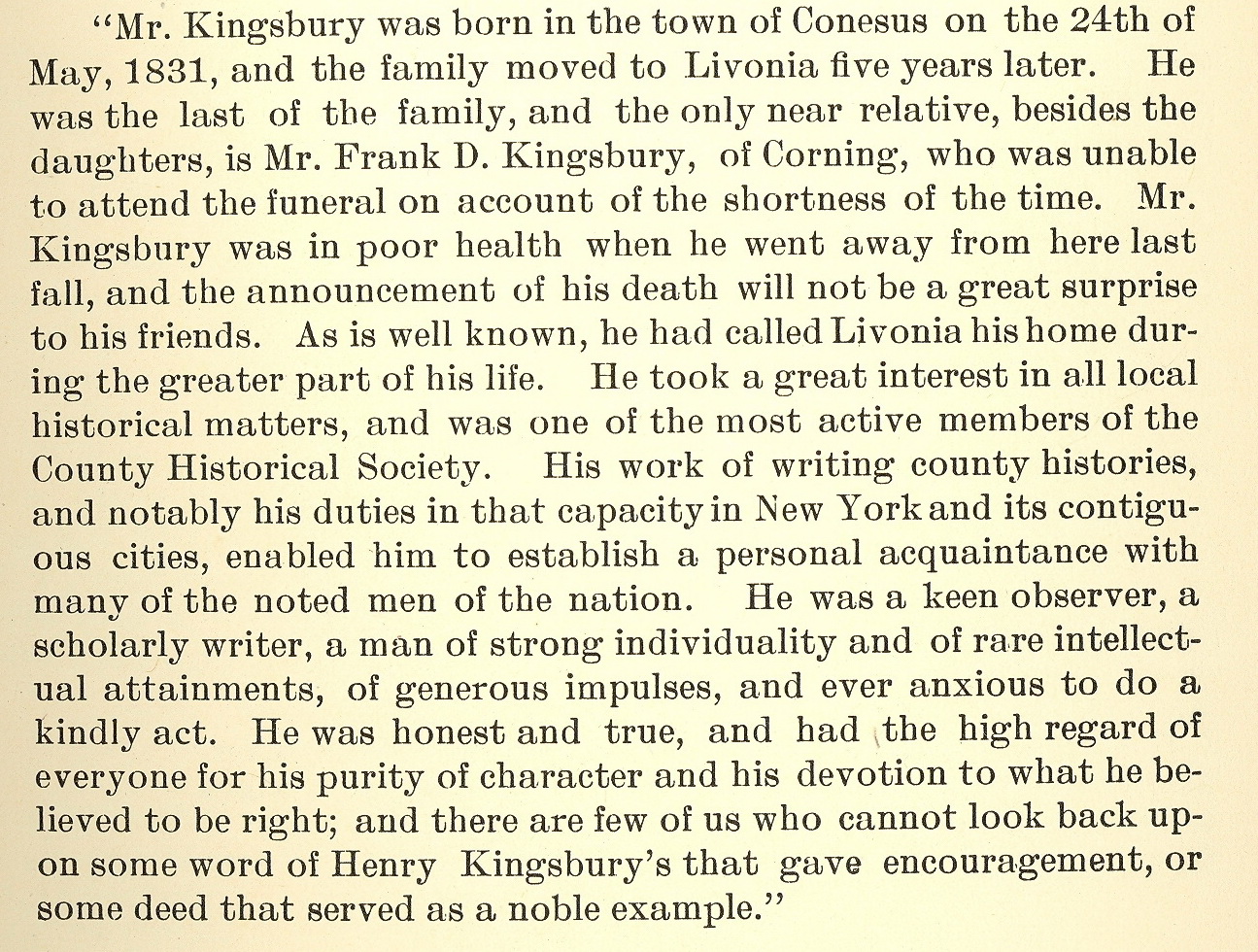This image is a sepia-toned excerpt from an old book or possibly a newspaper, providing an obituary for Mr. Henry Kingsbury. The text, printed in faint black font on yellowed paper, details Mr. Kingsbury's life and contributions. Born on May 24, 1831, in the town of Canesis, he relocated with his family to Livonia five years later. The obituary notes that he was the last surviving member of his immediate family, with Mr. Frank D. Kingsbury of Corning being the only near relative, who was unable to attend the funeral due to time constraints. Mr. Kingsbury had been in declining health since he left Livonia the previous fall, so his death did not come as a great surprise to his friends. Known for his profound interest in local history, he was an active and prominent member of the County Historical Society, making significant contributions through his scholarly writings on county histories in New York and its surrounding areas. His works allowed him to form personal connections with many notable figures across the nation. Described as a keen observer, a scholarly writer with strong individuality, and rare intellectual attainment, Mr. Kingsbury was also known for his generosity and integrity. He was highly regarded for his pure character and unwavering commitment to his beliefs. Many remember the encouragement he offered and his noble deeds, which served as an example to all.